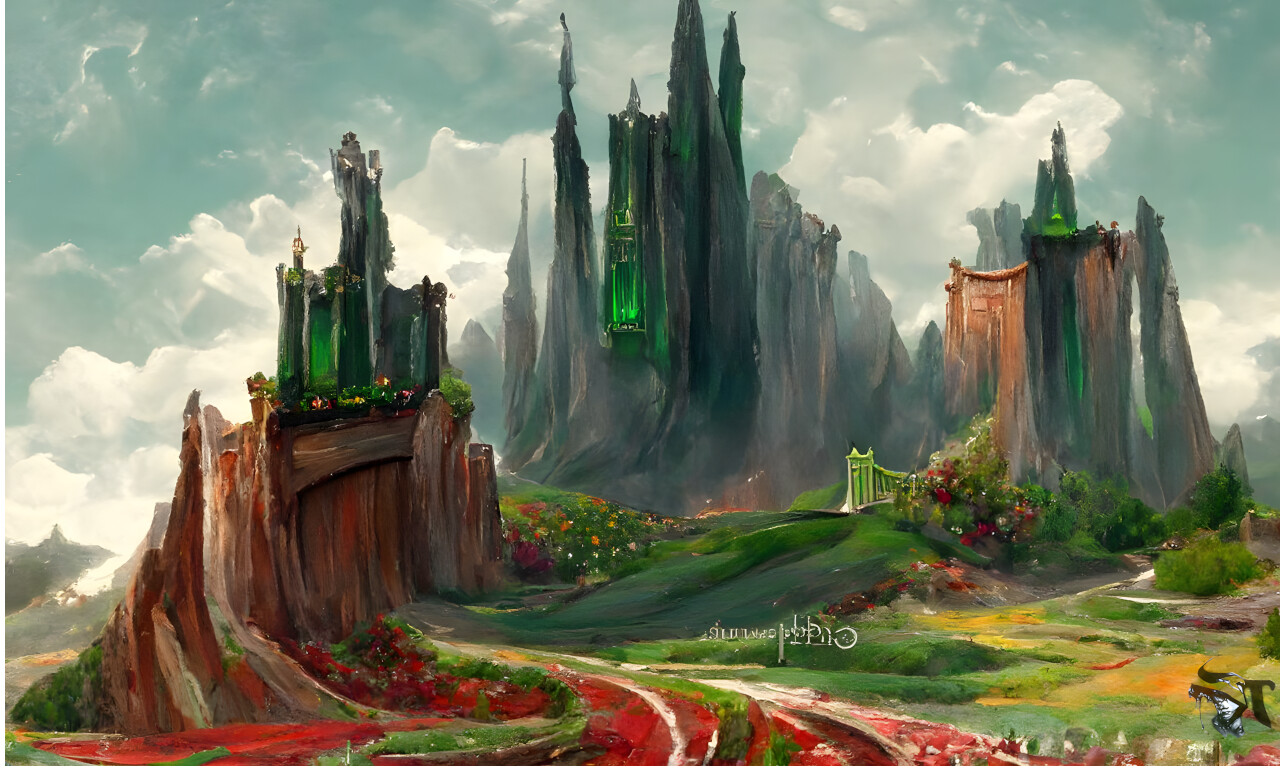This image is a vibrant, fantasy-esque painting, possibly created with watercolor or paint. It features a mystical landscape with three prominent, surrealistic castles atop green hills. The castles glow with emerald-like green light and have intricate details, including brown and red wooden doors and big steeples adorned with green crystal-like jewels. Each castle is set against a lush green valley decorated with vivid red, yellow, and orangey-pink flowers, providing a striking contrast to the backdrop of a cloudy sky with various shades of gray and white.

Towards the bottom middle-right of the image, there is an indistinct font or text, hinting at a potential connection to 'Lord of the Rings' though its exact meaning remains unclear. Paths adorned with red flowers wind through the landscape, leading up to the castles, enhancing the otherworldly and enchanting feel of the scene. The overall use of color—greens of the grass and castles, the diverse hues of the flowers, and the blue and white of the clouds—adds to the painting's captivating and magical atmosphere.